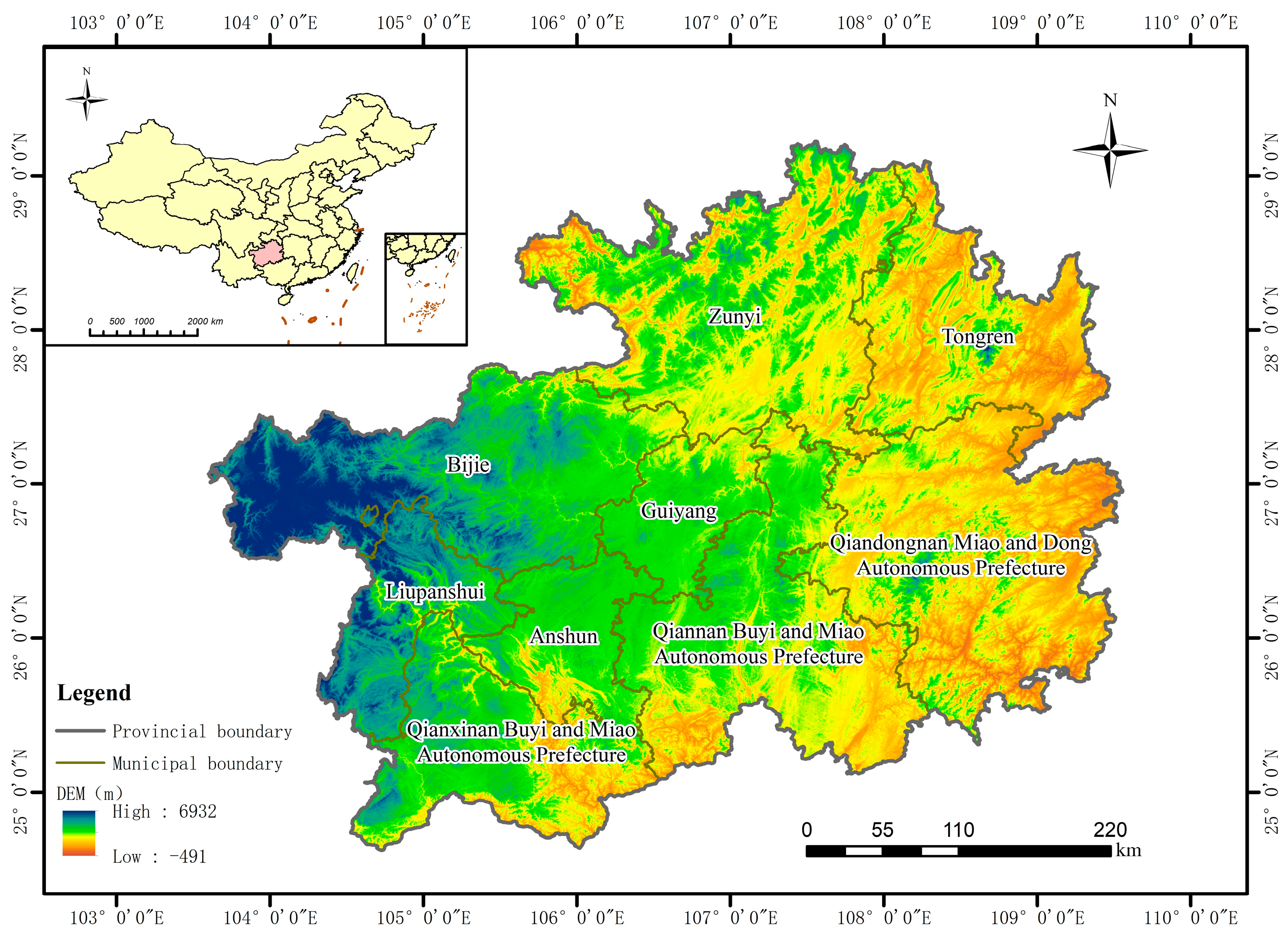This is a detailed colorful topographic map showcasing the elevation of several cities in a region of China. Elevation ranges from the lowest in red to the highest in deep blue. The left side of the map prominently features dark and light blues, indicating the highest elevations, while greens dominate the central area, and yellows, oranges, and reds signify lower elevations to the right and slightly above center towards the left. Cities such as Tongren, Bajai, and Gaiyang are marked, along with others, and the map includes provincial boundaries outlined in blue-gray and municipal boundaries in mustard yellow. Longitude and latitude indicators frame the map, with a compass pointing north in the top right corner. A legend in the bottom left explains the color scale (DEM in parentheses) and boundaries, and a small inset map highlights the specific Chinese region within the larger nation's context.